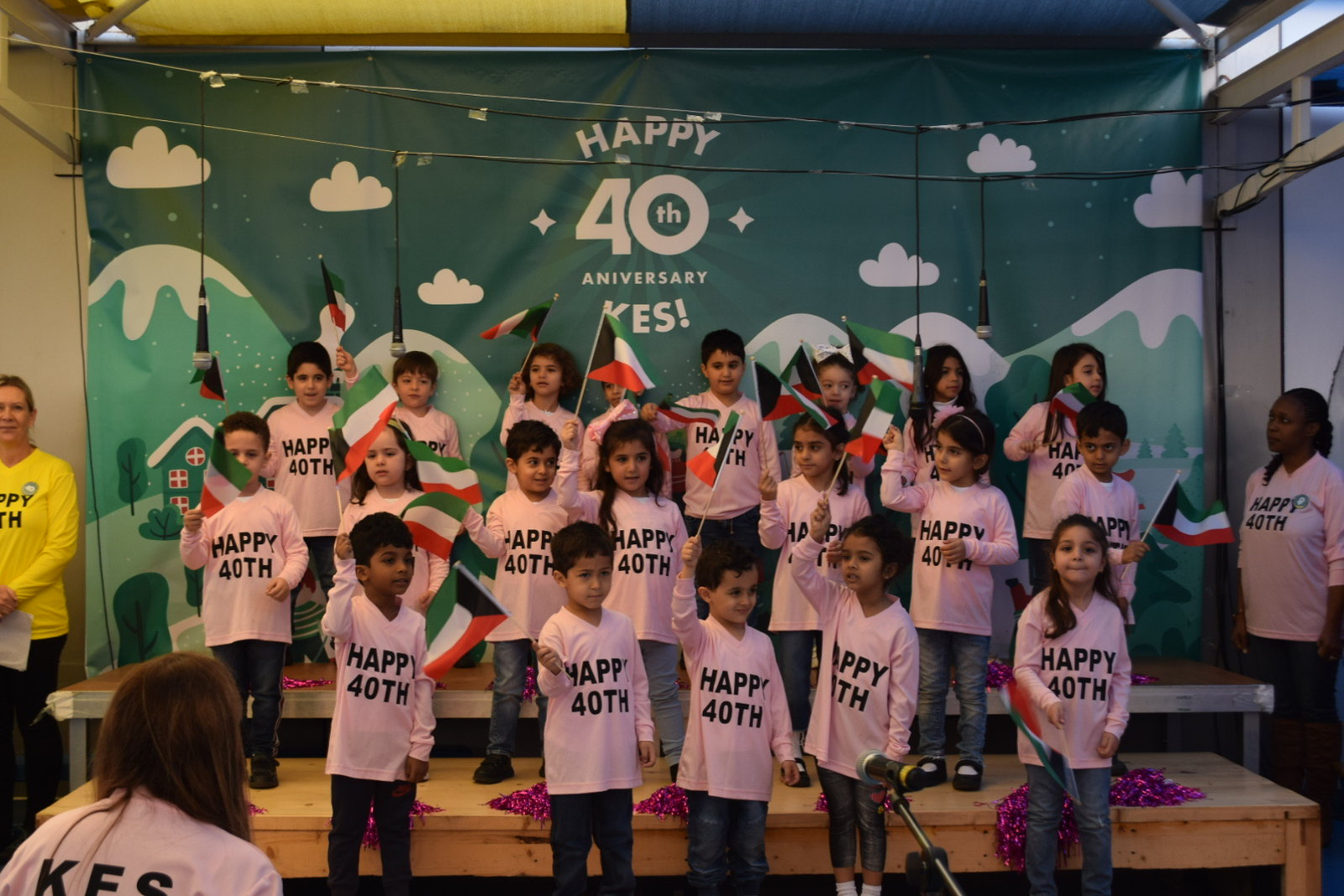The image depicts a lively and colorful indoor group scene featuring children and adults celebrating a milestone event. At the center of the photo, a group of children stands in front of a large green backdrop decorated with clouds, mountains, and the words "Happy 40th Anniversary" in bold white letters. The children, who appear to be part of a school class, are all dressed in matching pink long-sleeved shirts with "Happy 40th" printed in black text and are wearing black pants. They are joyfully holding up Palestinian flags. On the far left of the image, a white female teacher, wearing a yellow shirt also bearing the "Happy 40th" text, stands smiling, while on the far right, a black female teacher in a matching pink "Happy 40th" shirt joins the celebration. The bright and festive atmosphere, enhanced by the colorful banner and the children's cheerful expressions, suggests a joyous celebration of the school's 40th anniversary.